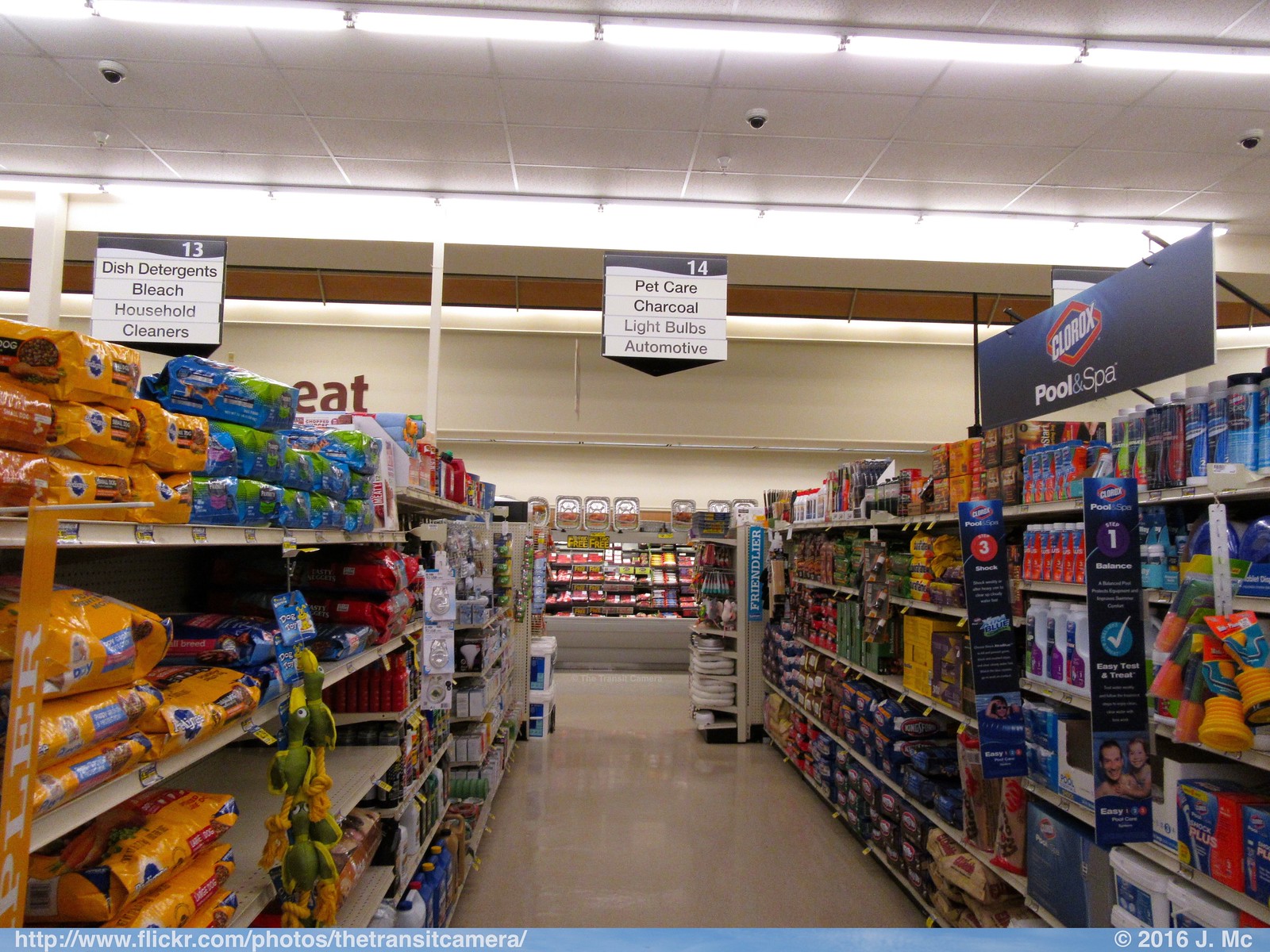This photograph captures aisle 14 inside a typical grocery store, displaying a well-lit, expansive space with a slick, beige flooring. The aisle is marked by a black-bordered sign hanging from the ceiling, displaying a white background with black letters that read "Pet Care, Charcoal, Light Bulbs, and Automotive." The ceiling features a grid of white tiles with long fluorescent lights running across, along with black half-globe security cameras.

On the left side of the aisle, there is a variety of dog foods, including brands like Pedigree and Alpo. As you move further down, light bulbs are displayed. Past these, the back of the aisle reveals sections of the meat counter and giant tinfoil roasting pans. 

On the right side, there are bags of charcoal and various automotive products such as oils and transmission fluids. Prominently, there is a Clorox Pool and Spa sign, black with white letters. Adjacent to aisle 14 is aisle 13, labeled with a similar sign indicating it contains dish detergents, bleach, household cleaners, and other cleaning supplies. Additionally, at the bottom of the image, a copyright note reads "© 2016 J.M.C." The URL http://www.flickr.com/photos/thetransitcamera/ is mentioned in the lower left corner.